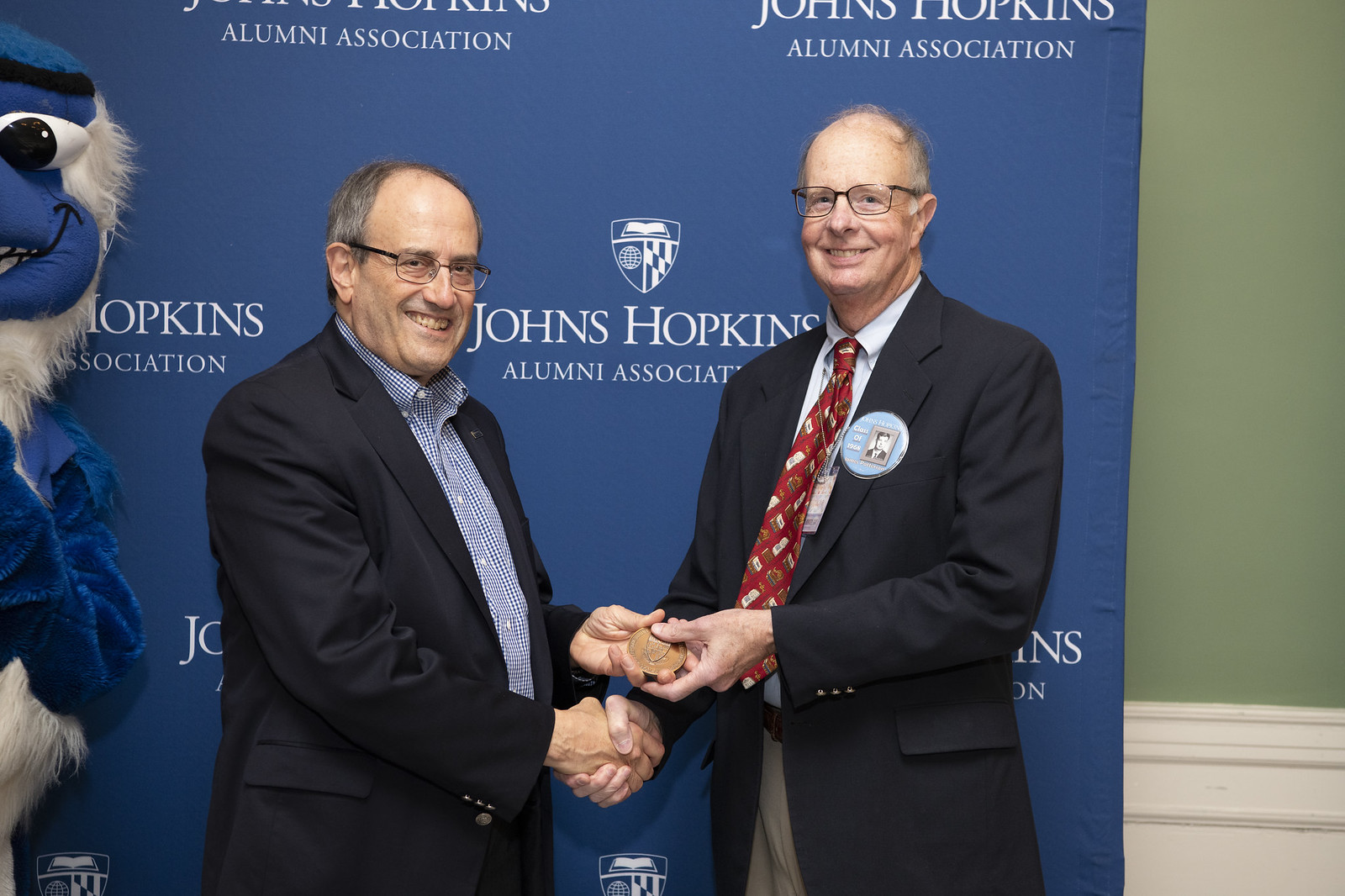In this indoor, photographic image set against a backdrop that reads "Johns Hopkins Alumni Association," two elderly white men are smiling and shaking hands while exchanging a gold-colored medal. Both men wear thin-rimmed glasses and have graying, balding hair. The man on the left, who has his shirt unbuttoned at the top and wears a blue and white striped dress shirt under a dark suit, holds the medal in his left hand. The man on the right, in a dark suit with a blue sports jacket, khaki pants, and a red patterned tie, clasps the medal with his left hand while also sporting a button featuring a child's photo. To the far left of the image, a partially visible blue and white duck mascot, likely for Johns Hopkins University, stands near a green wall, providing an additional hint of the celebratory setting.